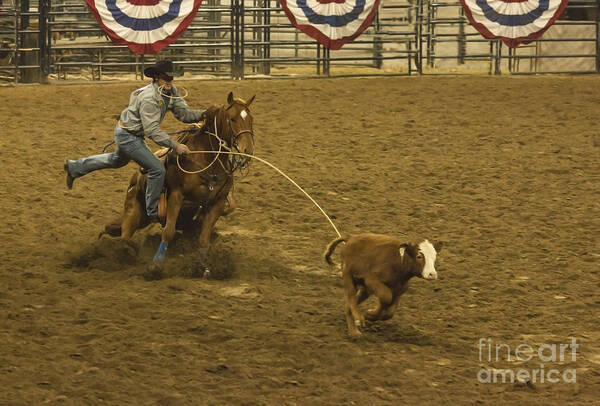The image captures an intense action shot at a Western rodeo event where a cowboy, dressed in a gray long sleeve shirt, blue jeans, and a black cowboy hat, is in mid-action of roping a calf. The cowboy, riding a brown horse with a distinctive white diamond on its forehead, is seen gripping a long tan rope aimed at a small brown calf that features a large white patch on its face. The scene unfolds in a brown, dirt-filled enclosed arena, scattered with hay, under the bright lights. The background reveals metal fences adorned with red, white, and blue bunting, adding a patriotic flair to the setting. The image also includes transparent white text at the bottom right that reads "Fine Art America."